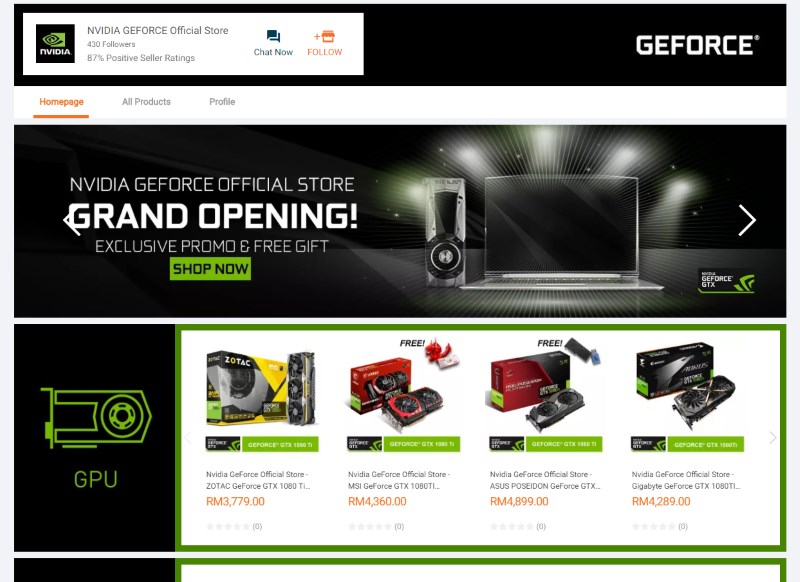The image depicts the homepage of an online store called the "NVIDIA GeForce Official Store." In the top left corner, there is a white background with black text that reads, "NVIDIA GeForce Official Store 1,000 daily followers 87% positive seller rating." Below this text, there are two buttons: a blue "Check Now" button on the left and an orange "Follow" button on the right. The NVIDIA logo, featuring a black emblem with a green eye and the word "NVIDIA," is also present in the top left corner.

On the top right, white text on a black background spells out "GeForce." Below, the main navigation menu is divided into three tabs located at the top left: "Home Page," "All Products," and "Profile." The "Home Page" tab is highlighted in orange, indicating it is the current active page, while the other tabs are in gray.

The central section of the homepage features a promotional banner with a black background. On the left side of this banner, white text announces the "NVIDIA GeForce Official Store Grand Opening Exclusive Promo and Free Gift." Below this text is a green "Shop Now" button. On the right side of the banner, there are images of a laptop and a gray graphic card, accompanied by the text "NVIDIA GeForce GTX."

Directly below the banner, the left side features green text that reads "GPU" alongside a green drawing of a GPU. On the right side, there are four listings for different graphics cards, each with a white background. The products include:

1. **NVIDIA GeForce Zotac GeForce GTX 1080Ti** - priced at RM 3779.00
2. **MSI GeForce GTX 1080Ti** - priced at RM 4360.00
3. **ASUS Poseidon GeForce** - priced at RM 4899.00
4. **Gigabyte GeForce GTX 1080Ti** - priced at RM 4289.00

The product names are written in black text, while the prices are highlighted in orange.